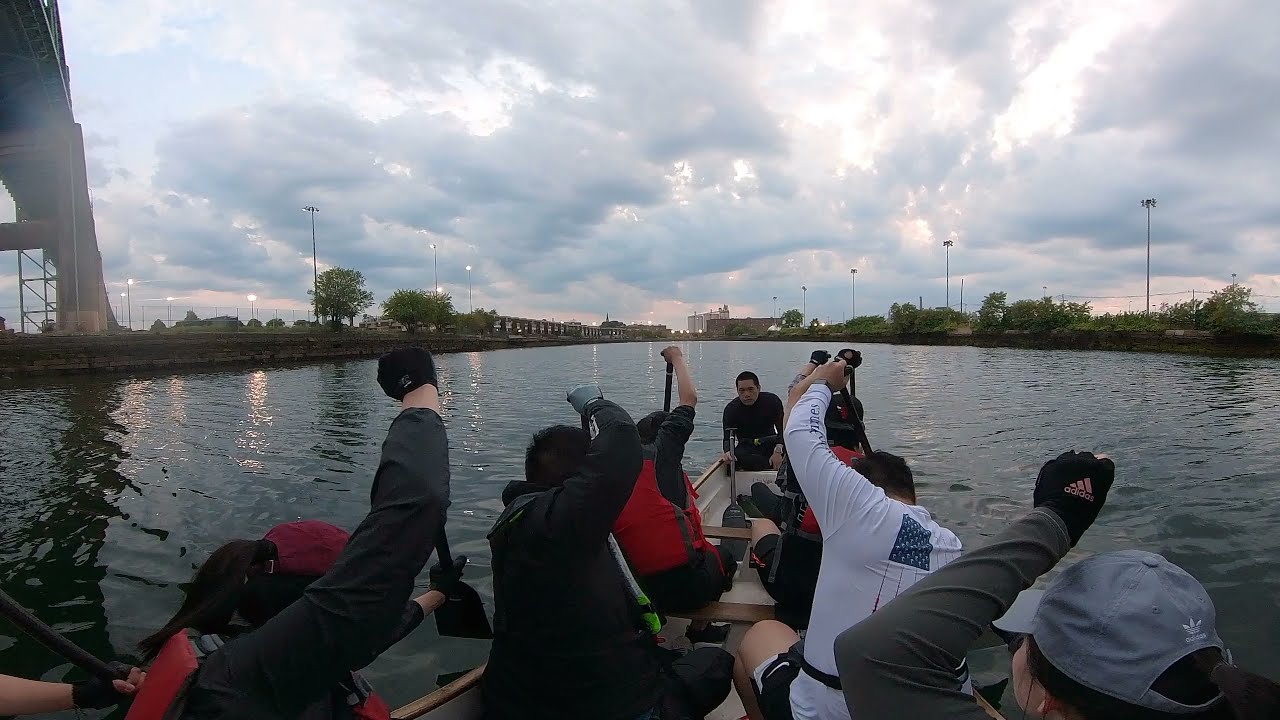This image captures a group of nine people, possibly Asian, in a long, canoe-like boat navigating through a dark waterway that could be a river or canal. It's either early morning or late afternoon, suggested by the cloudy sky tinged with hues of purple and pink, and the sun peeking through the clouds. In the foreground, a trestle or bridge spans the waterway, enhancing the urban atmosphere of the scene. The boaters, clad in jackets and gloves indicating chilly weather, display camaraderie with fists raised in different motions. Their attire varies from dark tops to a distinctive black top with a red life jacket, and a white top seen on one individual. The head of the boat features a person facing the crew, possibly the leader. Surrounding the body of water are shorelines dotted with bushes, trees, and tall lampposts, and distant city buildings further assert the scene’s metropolitan setting. Notes of particular details such as a Chicago Bulls hat hint at a potential geographic location near Chicago.